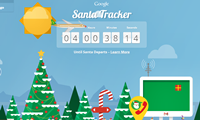This image features the Google Santa Tracker, a festive, Christmas-themed interactive software that allows users to follow Santa Claus as he travels around the world on Christmas Eve. The primary focus at the top of the image is a countdown timer, prominently displaying the time remaining until Santa's departure, which currently reads 4 hours, 38 minutes, and 14 seconds. Above the countdown, the word "Google" is clearly visible, while "Santa Tracker" is written below in an interesting and whimsical font.

The overall theme is adorned with a blue background, decorated with fluffy clouds, a few mountains, Christmas trees, and a candy cane. A prominent sun is situated in the upper left-hand corner, serving as the focal point of the image without any additional icons. There is also a small gift icon hinting at interactive elements within the tracker, potentially allowing users to engage further with the software. The entire scene creates a cheerful and vibrant holiday atmosphere, effectively capturing the spirit of Christmas.